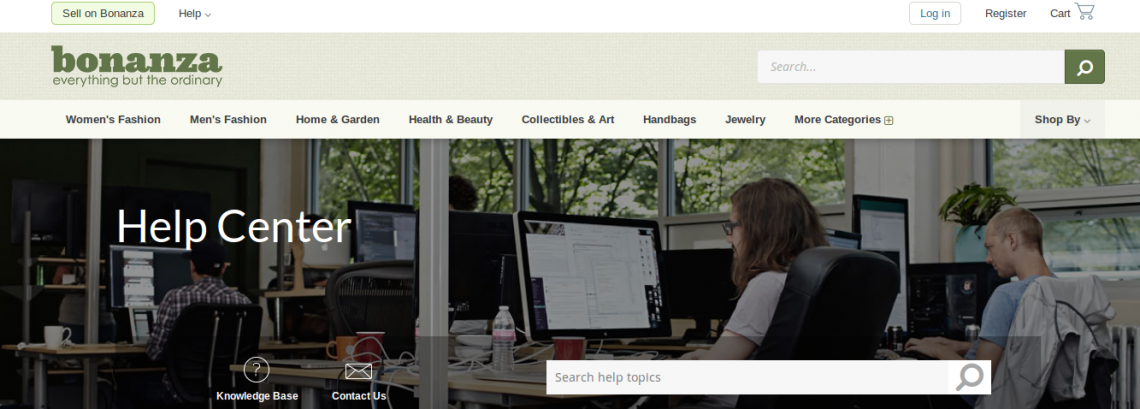The image is a detailed screen capture of Bonanza’s website interface, showcasing its branding and navigation elements alongside a visual glimpse into its help center. At the top center, the Bonanza logo is prominently displayed with the company motto, "Everything but the ordinary," just below it. Above the logo, a vibrant green button labeled "Sell on Bonanza" catches the eye, accompanied by a help drop-down menu.

On the far right, user options such as "Login" are presented in blue letters encircled, with "Register" and a shopping cart icon adjacent to them. A search bar with a magnifying glass icon set against a dark green background is positioned towards the right end of the same top bar.

Beneath the Bonanza logo and menu bar, an array of category links spans from left to right, including "Women's Fashions," "Men's Fashions," "Home and Garden," "Health and Beauty," "Collectibles and Art," "Handbags," "Jewelry," "More Categories," and a "Shop by" menu indicated by an arrow for further navigation options.

Dominating the lower part of the screen is an image depicting Bonanza's help center office environment. Here, several employees are engaged in their work at flat-screen computer monitors. Central to this image is a young woman with long, medium brown hair and dark glasses, dressed in a white short-sleeved top. Beside her, a man with a mostly shaved head and a blue short-sleeved shirt is focused on his keyboard. On the left side of the picture, another man, clad in a long-sleeved plaid shirt of various shades of brown, white, and black, also works diligently at his computer.

The desks are cluttered with typical office paraphernalia like coffee cups, mugs, water bottles, and visible wiring. At the bottom of the image are interactive buttons labeled "Knowledge Base" with a question mark icon, "Contact Us" featuring an email icon, and a search bar for selecting help topics, completing the professional yet approachable atmosphere of Bonanza’s customer service interface.